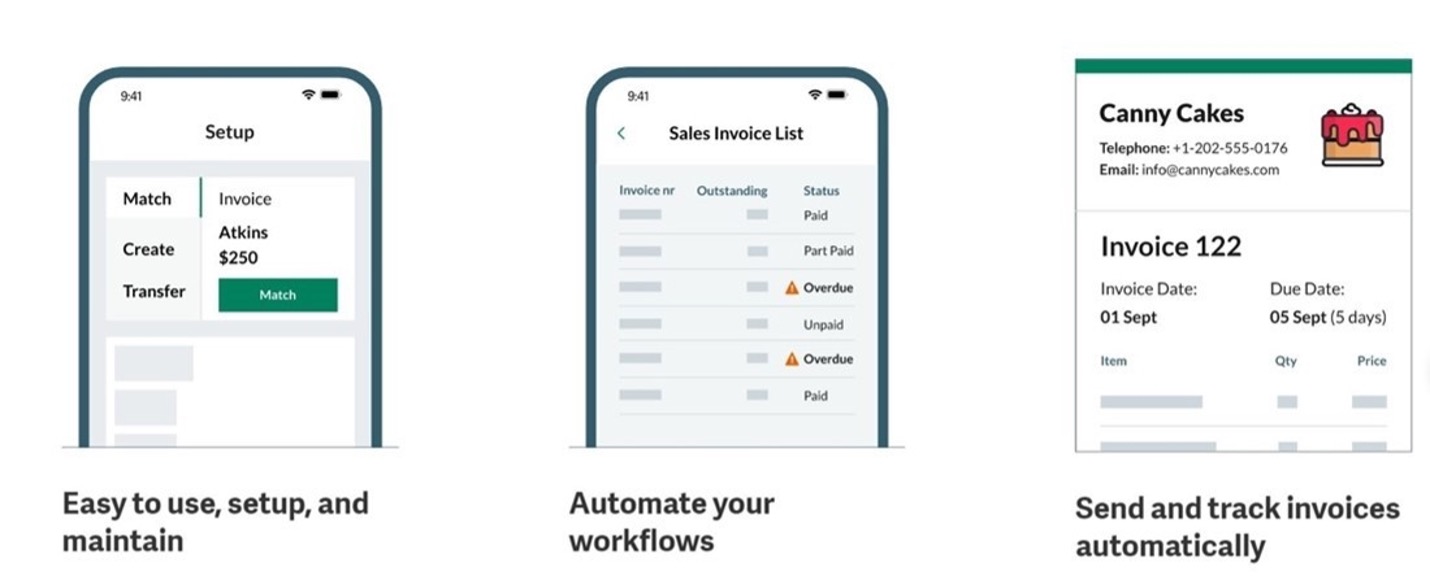A detailed mock-up showcases various smartphones with intricate designs and specific interface elements. The smartphone on the left features a dark blue bezel. The top left of the screen displays "9:41" in white, centered is the bold black text "Set Up," and on the right side are black icons for Wi-Fi and battery status. Moving down, a gray section contains two stacked rectangles; the left one reads "Match," "Create," "Transfer," and the right one presents an invoice. Below, in bold black, it lists "Atkins," priced at $250. A dark green rectangle in the center has "Match" written in white. Underneath, it is labeled in bold black as "Easy to use, set up, and maintain."

Central to the image is another smartphone mock-up with a similarly dark blue bezel showing "9:41" at the top left. A teal arrow directs attention leftwards, highlighted by the bold black text "Sales Invoice List." The screen contains gray placeholders for content, with headings in blue: "Invoice Nr," "Outstanding," and "Status." Several statuses are identified: "Paid," "Part Paid," an orange triangle with an 'I' indicating "Overdue," "Unpaid" in gray, "Overdue" again in bold black with the triangle, followed by "Paid." The text "Automate Your Workflows" appears in bold black.

A section towards the right highlights a web page mock-up banner in green titled "Candy Cakes" in bold black, featuring an image of a brown and tan cake with red dripping icing, red fruit pieces, and a white frosting curl on top. Details include contact information, with "Telephone" in bold black formatted as "+1-202-555-0176," and "Email" as "info@candycakes.com." An invoice labeled "Invoice 122" provides further specifics: "Invoice Date - 01 SEPT" and "Due Date - 05 SEPT (5 days)." Several dark gray rectangles list items under headings in blue: "Item," "QTY," and "Price."